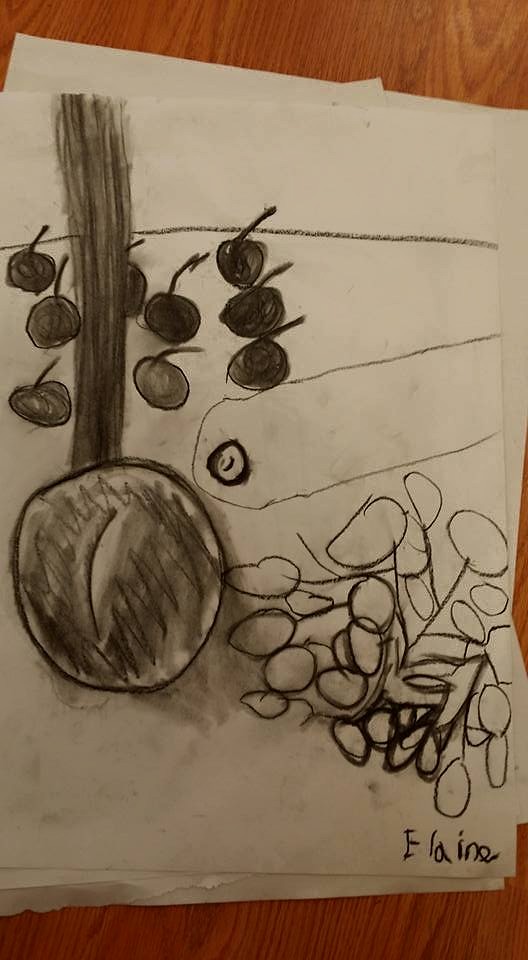The photograph captures a drawing on a white A4 piece of paper, which is part of a larger stack of papers. This stack is placed on a wooden table with a varnished surface, giving the wood a honey-toned appearance. The table, possibly made of pine or oak, displays visible planks and an intricate wood grain pattern that is noticeable both at the top and bottom of the image. The photograph was taken indoors under an overhead light, resulting in a somewhat dim overall ambiance.

The drawing itself seems to be a child's work, suggested by its simplistic and whimsical style. The name "Elaine" is handwritten in plain, non-cursive script in the bottom right corner of the paper. Rendered in black charcoal, the drawing features a large fruit, perhaps a pear, on the left-hand side with an elongated stalk extending to the top of the page. Nine smaller fruits are clustered behind the stalk. On the right-hand side, two horizontal lines converge to form a shape reminiscent of a carrot. Above the name "Elaine," there is a depiction that resembles a bunch of grapes. The entire composition feels playful yet unpolished, encapsulating the charming essence of juvenile creativity.